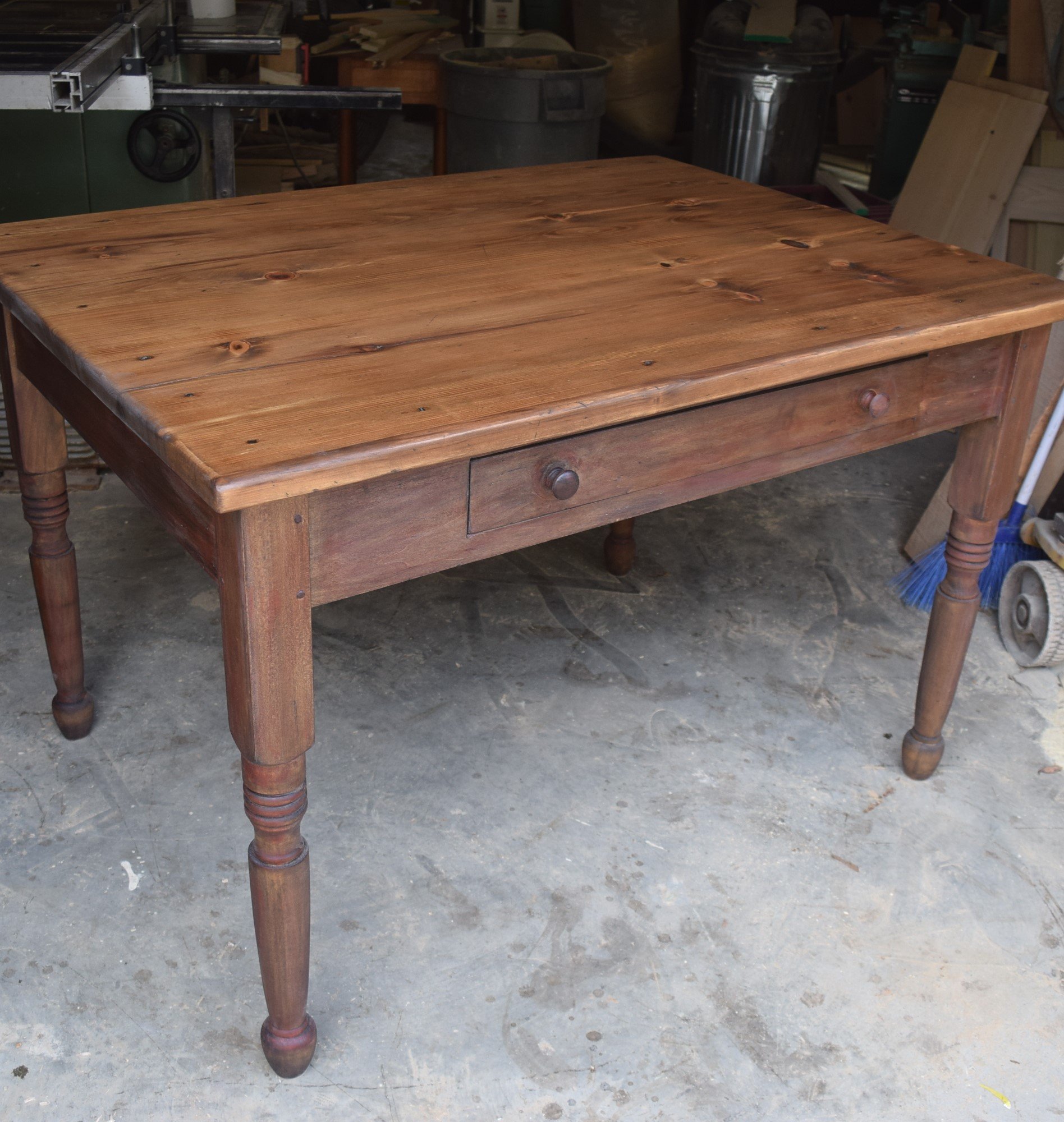The image depicts a vintage, medium-brown wooden table with a greenish hue, positioned in a cluttered garage. The table, which appears to be in good condition despite some scuffs along the edges and legs, features four legs and a front drawer with two knobs. The garage has a gray, dusty concrete floor marked by drag lines. In the background, there is an assortment of items, including a shelving unit, a chair, stacks of wood slabs, a green box, and both a gray plastic and a silver metal trash can. Additionally, a broom is visible to the right, and the upper left is filled with a metal frame and other piled-up items. This detailed scene suggests the table may be prepped for repurposing or sale.